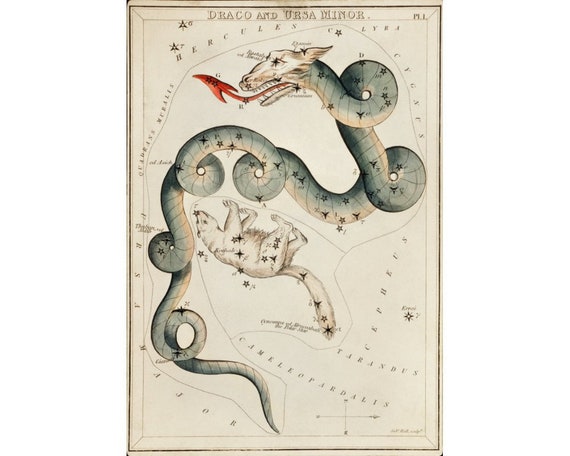This detailed star chart illustration, crafted on vintage beige-gray paper, showcases the constellations Draco and Ursa Minor, as indicated by the title at the top. Framed by a dark brown border with intricate, indented corners accentuated by a fainter brown inner line, the artwork depicts an elaborate dragon entwined with numerous loops and bends, symbolically mapping stars along its serpentine body. The dragon, characterized by a yellow-red forked tongue flicking to the left and a visually striking cross on its eye, appears animated with a slightly whimsical, almost dog-like head with ears. Below the dragon, a pale white bear with an unusually long tail, depicting Ursa Minor, adds to the celestial narrative. Additional star formations, including Hercules and Lyra, enrich this unique and meticulously detailed poster, reminiscent of old-fashioned celestial maps that blend mythology with stellar cartography.